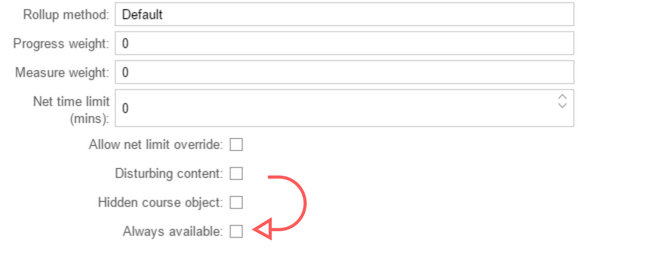This screenshot from the Rollup app displays the user interface requesting details for the user's Rollup method, which is set as "Default." The user has entered "0" for both their progress weight and measure weight, and has also set the net time limits to "0 minutes." At the bottom of the interface, four options are available: "Allow Net Limit Override," "Disturbing Content," "Hidden Course Object," and "Always Available." A red, curved arrow points from "Disturbing Content" to "Always Available," indicating some relationship or transition between these options. No additional content has been provided at this stage.